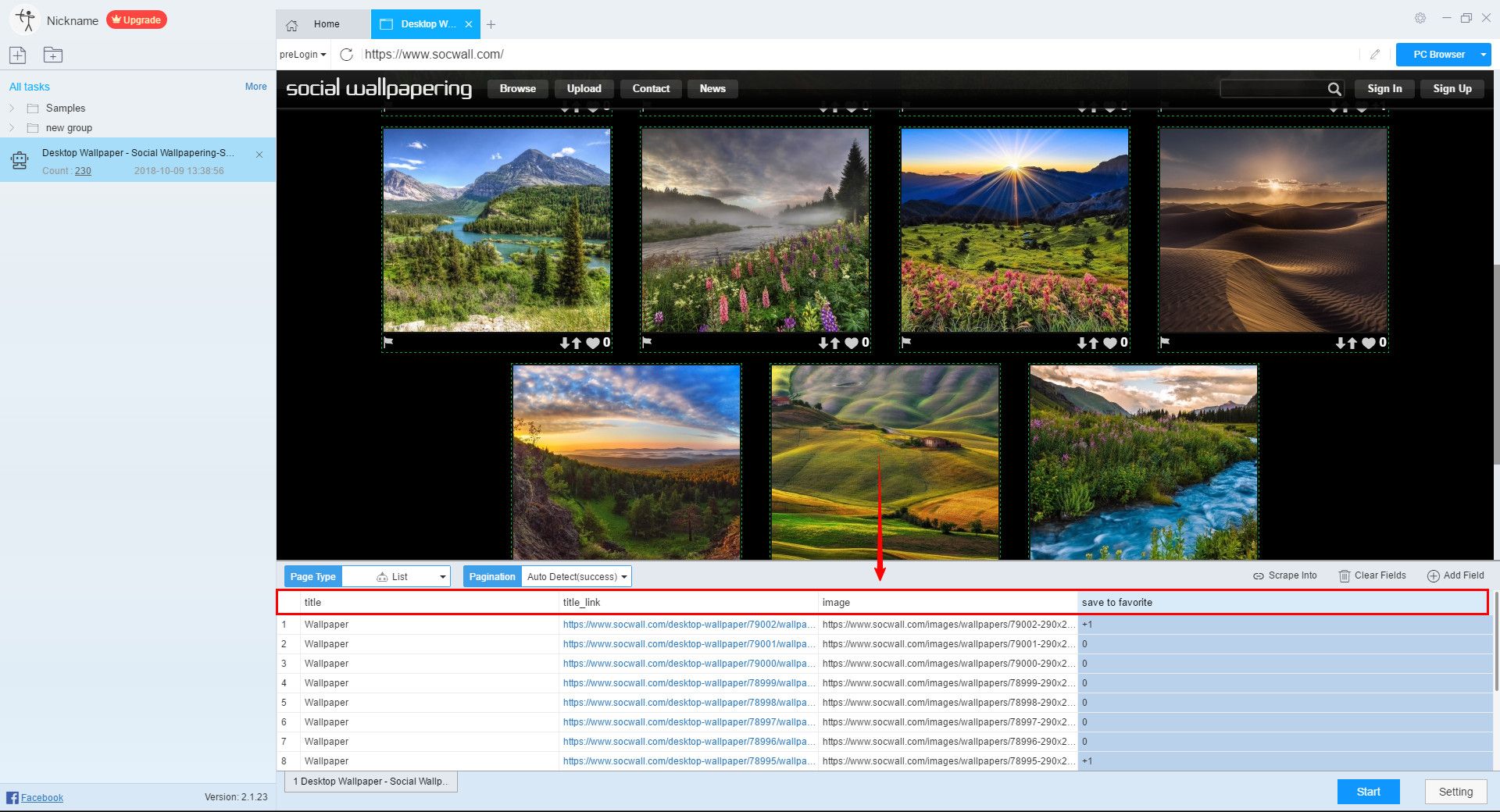A detailed screenshot of an automated social media posting program interface. On the top left, a file tree is visible with a highlighted section featuring a robot icon, indicating the active or selected component. To the right, a series of thumbnails showcasing various nature views are displayed prominently. At the bottom center, a red arrow points downward, drawing attention to a highlighted top line within a lower section. This section contains lists of files, their names, links, and descriptions. The category headers at the top of this box are emphasized with a red rectangle. The highlights and annotations likely serve to demonstrate tagging or automation features. While the text within the interface is too small to read, the visual elements and layout are distinctly legible.